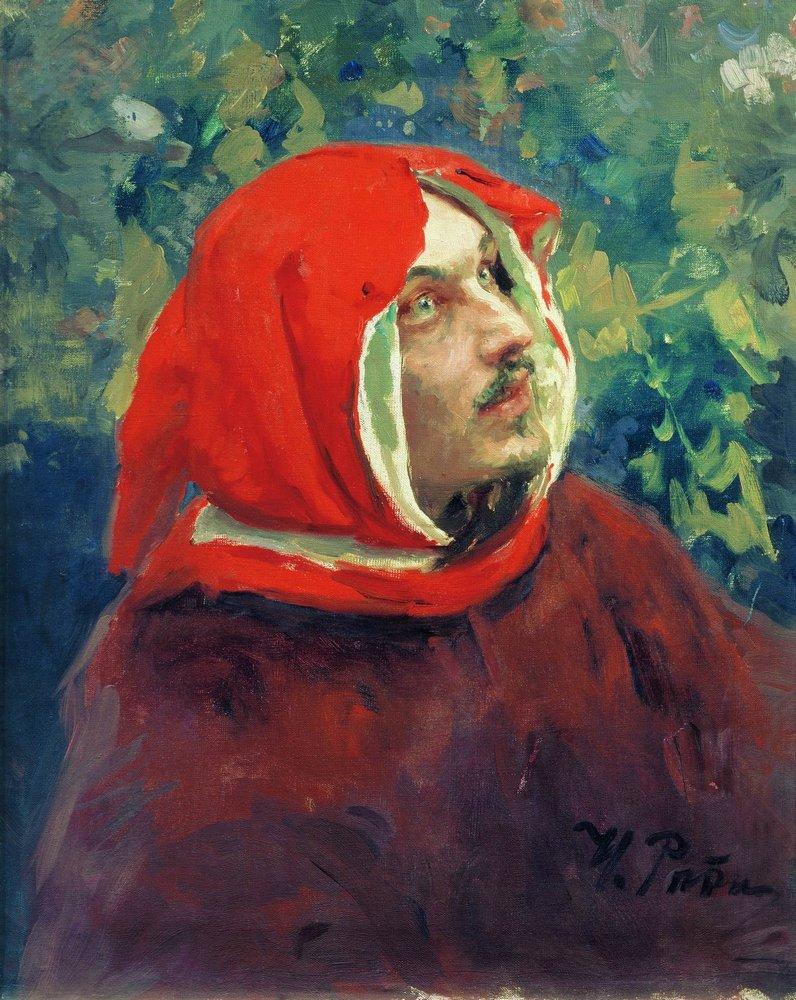This detailed color oil painting titled *Portrait of Dante Alighieri, 1265-1321*, created by Ilya Repin, captures an iconic image of the famed Italian poet. The painting is executed in a realistic style with prominent brush strokes. Dante is depicted in the lower center of the portrait, filling approximately two-thirds of the frame. Wearing a red robe and a distinctive headscarf that is red with a cream-colored lining, he gazes upwards towards the top right corner with raised eyebrows, a hint of a smile, and light green eyes. Dante's facial features include a dark mustache and a goatee beard, giving him an appearance that suggests he is in his 40s to 50s. The background features stylistic green leaves and a bluish area which might represent a wall. The artist's large signature is visible in the bottom right corner, with some letters discernible like "Y" and "P." The composition evokes a sense of awe and reverence, possibly alluding to Dante's religious affiliation, likely Catholic.